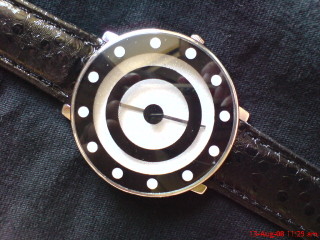This photograph showcases an elegant watch artistically placed on a blue cloth backdrop. The watch features a sophisticated brown leather wristband that complements its overall design. The face of the watch is characterized by a minimalist approach, with a sleek black outer circle adorned with white dots in place of traditional numerals. Moving inward, the dial is composed of alternating circles: a white stripe, a thin black stripe, another white stripe, and finally, a central black dot. The silver hour and minute hands, designed with a refined simplicity, indicate the time as 8:12.